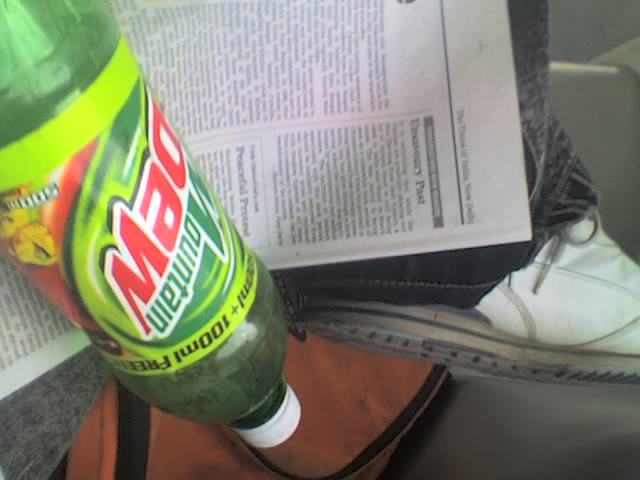This color photograph features a close-up of an upside-down plastic Mountain Dew bottle situated to the left, displaying the old logo where "Mountain" is fully spelled out. The bottle's white cap rests on a brown surface, likely part of a chair, and its green plastic exterior contrasts with the detailed label: "Mountain" in green, "Dew" in red on a white background, with that white set against a green backdrop adorned with darker green swirls. The bottle is positioned against a black and white newspaper, which is mostly in view but the text is unreadable due to blur and small newsprint. To the right of the newspaper, the photograph reveals the lower portion of a person - their dark, blackish-gray pant leg, white sneaker with visible gray shoelaces, and the chair beneath, suggesting a casual, seated position.